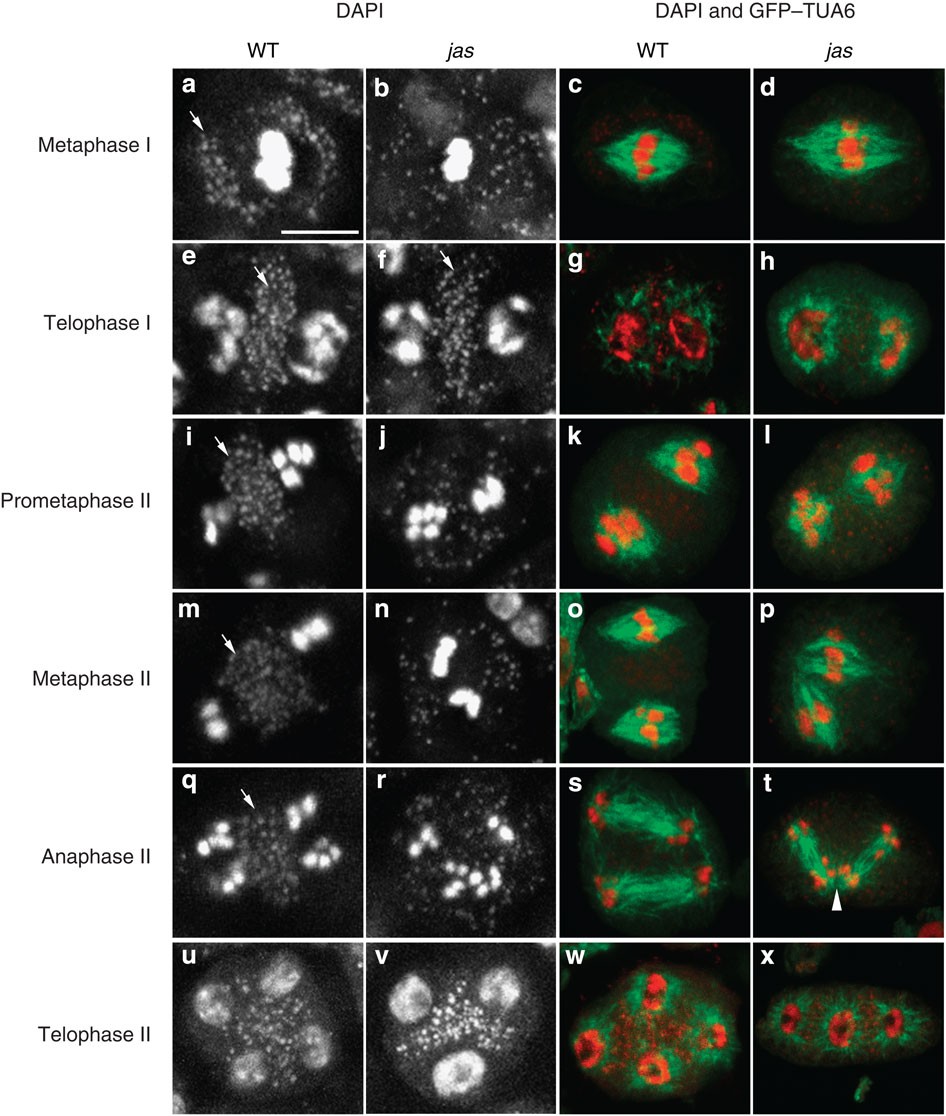This detailed scientific diagram consists of 24 microscope slide images arranged into four columns and six rows, with clear labeling along the top and left sides. The top labels read 'DAPI' for the first two columns and 'DAPI and GFP-TUA6' for the third and fourth columns. The first two columns display images in black and white, while the third and fourth columns feature images in red, green, and black, set against a black background. Each row represents different phases of cell division: metaphase 1, telophase 1, prometaphase 2, metaphase 2, anaphase 2, and telophase 2. Both halves of the diagram are vertically separated, showcasing an intricate examination of cells or organic material, with the colorized images highlighting a multiplying red substance. Additionally, the left side bears labels from A to X, identifying each individual slide.